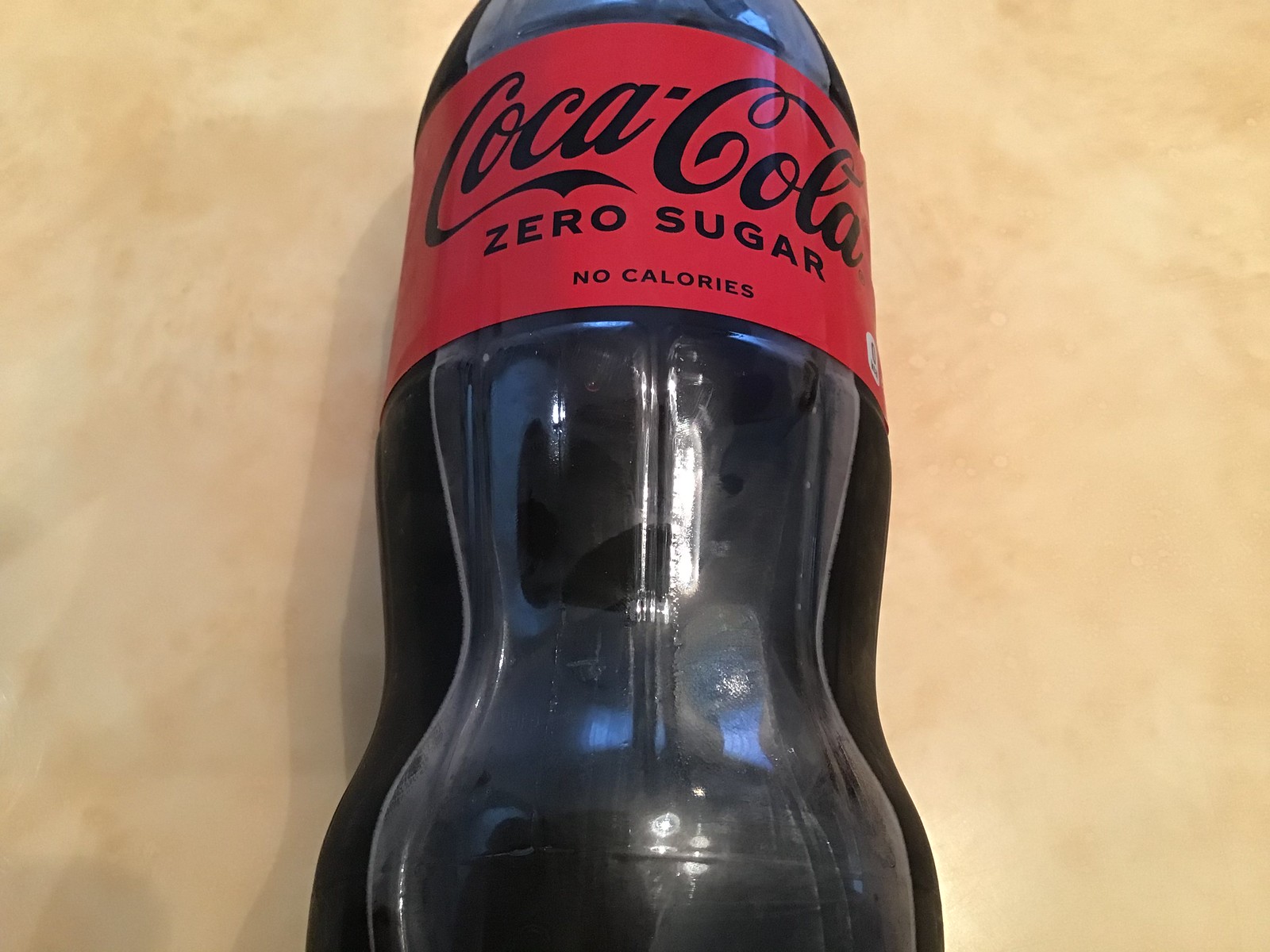This close-up photograph depicts a Coca-Cola Zero Sugar bottle lying on its side against a beige, tabletop-like background. The plastic bottle features a red label at the top with the black text reading "Coca-Cola Zero Sugar No Calories." The bottle is modeled after the classic Coca-Cola glass bottles, with a contour that dips inward slightly before expanding back out towards the bottom. The light source behind the camera causes reflections on the bottle's surface. A small white spot on the bottom right side of the red label contains some illegible writing, likely nutritional information. The bottle appears to still contain the product.